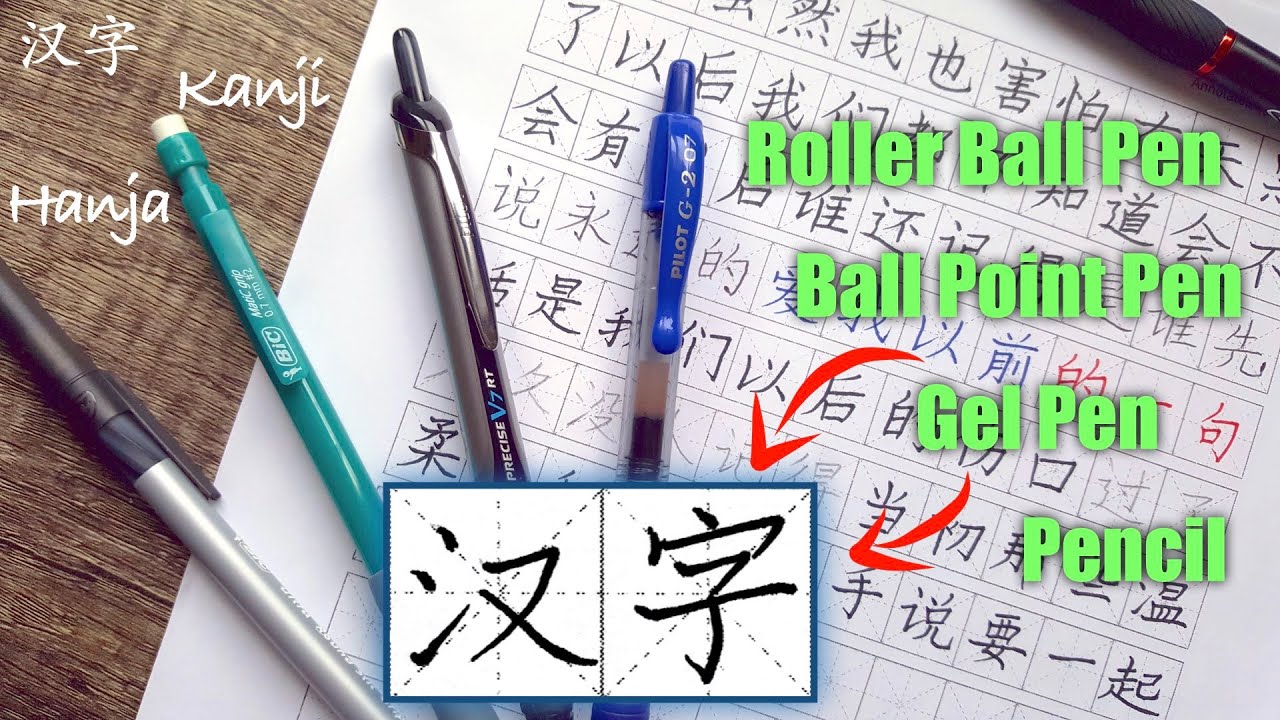The horizontal rectangular advertisement showcases four distinctive writing instruments—highlighting the variety of markings they can create. Prominently, on the right side in bold, large, lime-green letters, it lists: "rollerball pen, ballpoint pen, gel pen, and pencil." The four pens include a silver pen with a black cap, a turquoise pen, a brown pen, and a clear pen with a blue top. The central part of the image features two squares containing oriental characters, labeled with directional text pointers. These characters, set against a backdrop that suggests the intricate beauty of Chinese or Japanese calligraphy, exemplify the precision and art that can be achieved with these writing tools. The wooden surface underlying all the elements adds a touch of warmth and sophistication to the advertisement.